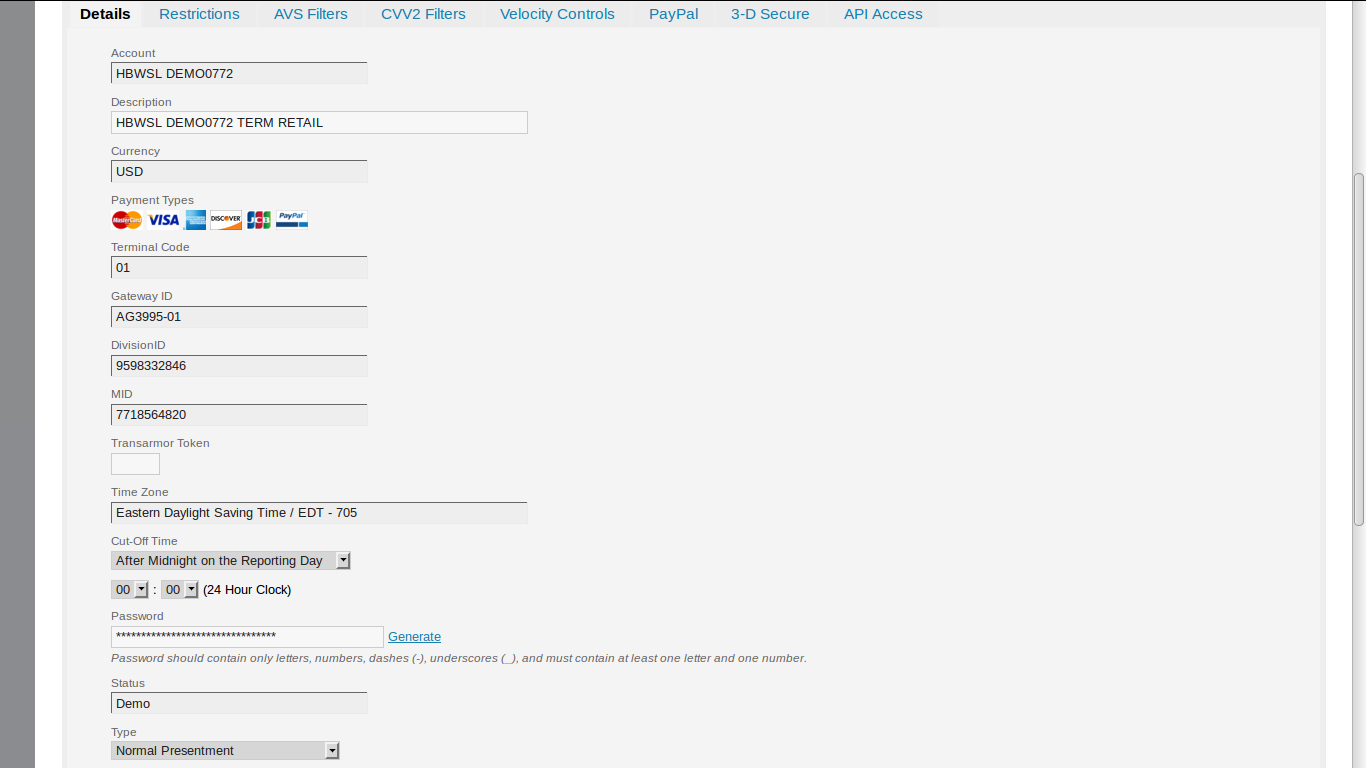A screenshot from a website displaying the payment type section of the checkout process. The screen shows that the user is approximately halfway down the page, indicated by the scrollbar on the right side. Across the top of the image, there are several categories in blue text, except for the first one in black, signifying the current selection. The categories listed are: Details, Restrictions, AVS Filters, CVV2 Filters, Velocity Controls, PayPal, 3D Secure, and API Access.

The page is currently on the "Details" section, requesting typical payment information such as account description and currency type. It also displays logos for various payment methods, including MasterCard, Visa, American Express, Discover, JCB, and PayPal. Below this, the section includes fields for Terminal Code, Gateway ID, Division ID, MID, TransArmor Token, Time Zone, Cutoff Time, Password Status, and Type, all in black font.

On the left-hand side of the image, there is a gray bar and a white bar providing structural border division.